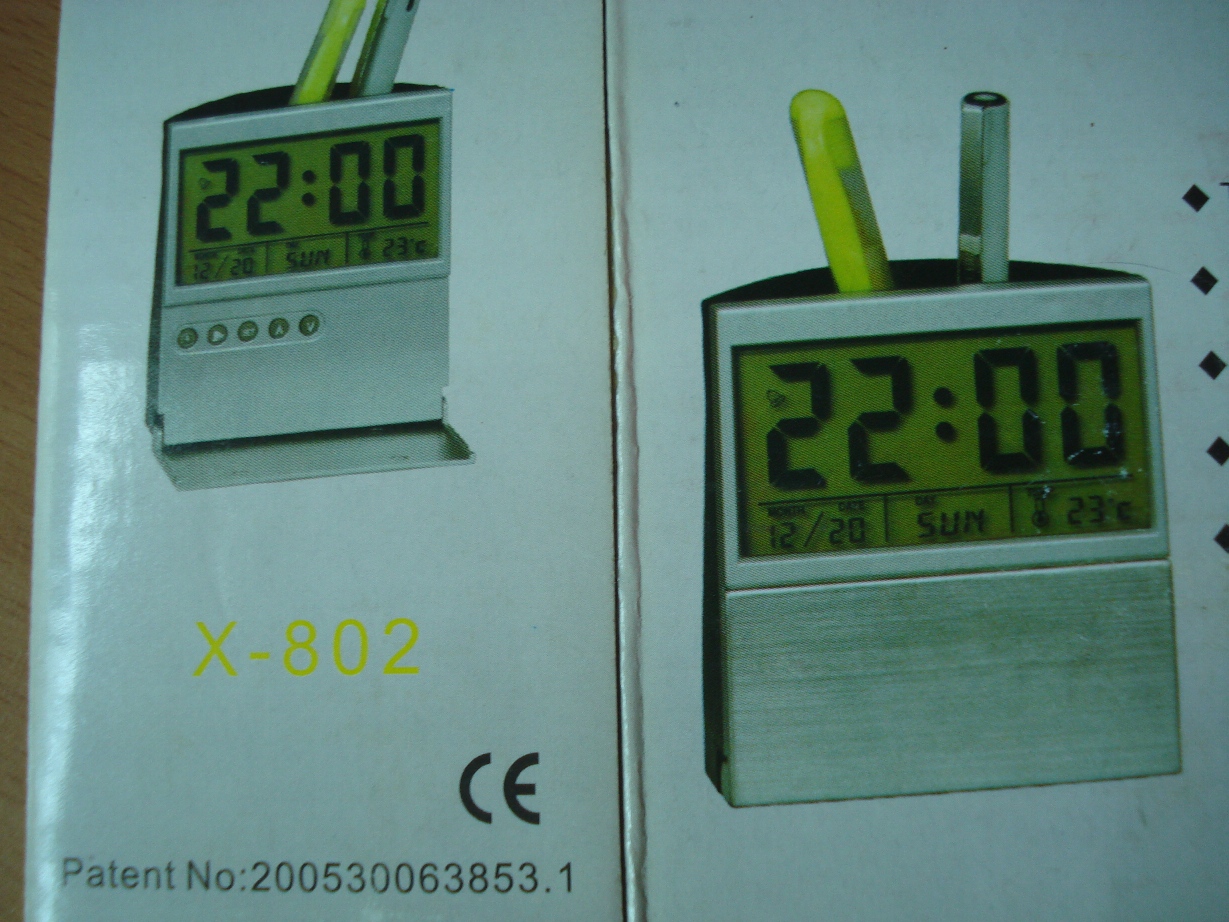The image features two digital timepieces mounted on what appears to be a plastic-coated sheet of paper. Each timepiece includes small compartments resembling pen holders. The timepiece on the left displays a patent number, "20053-00638531," along the bottom left corner, with the model number "X-802" situated above it, and the initials "CE" placed between these two sets of numbers. Both timepieces are synchronized, showing the same time, "22:00," and date. However, the timepiece on the right is noticeably larger than the one on the left. This setup seems to be for a scientific or technical purpose, potentially used for monitoring or recording data, suggested by the presence of pen-like instruments embedded in the clocks.